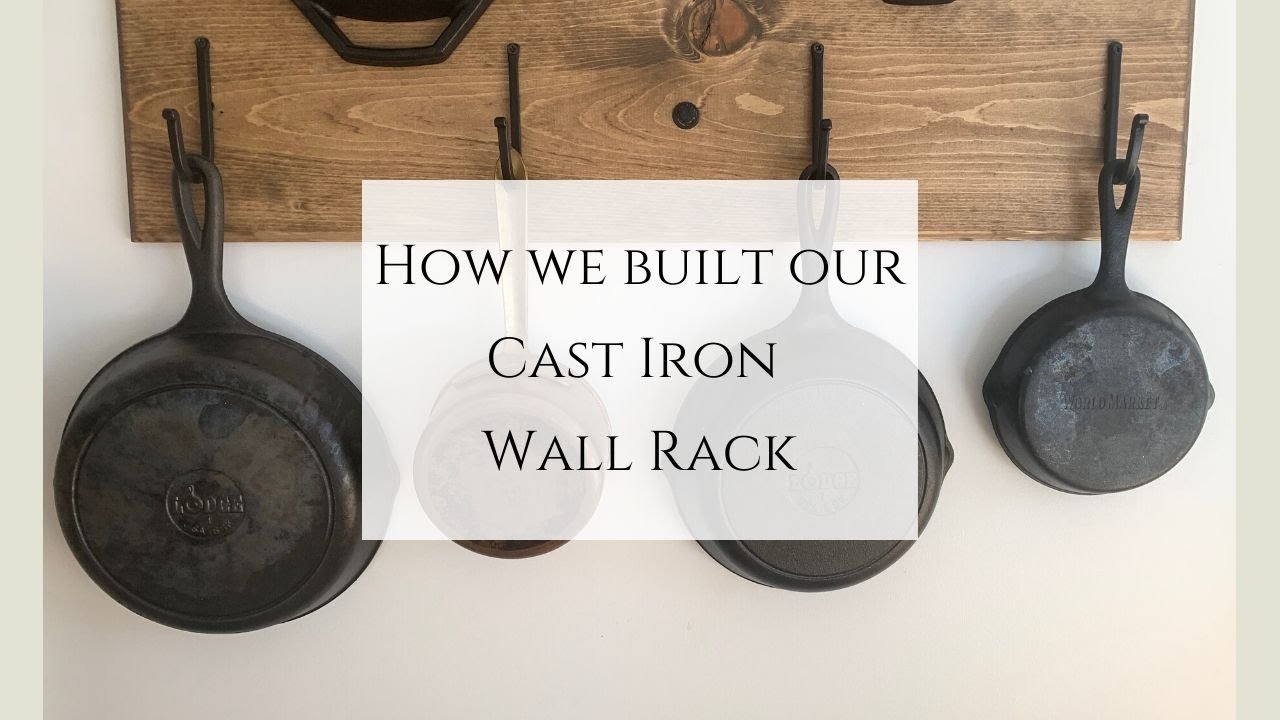The image showcases a DIY cast iron wall rack, ideal for home cooks and enthusiasts looking for practical kitchen storage solutions. The rack is a wide, light brown stained wooden plank mounted on a typical white painted wall. It features four sturdy iron hooks from which various sizes of cast iron skillets hang. The hooks support an array of pans: the largest on the left, transitioning to a smaller skillet, a medium-sized pot, and another skillet on the right. Overlaid on the middle of the image is a semi-transparent, rectangular white banner with black text in Times New Roman font that reads, "How we built our cast iron wall rack." The sleek black surfaces of the cast iron pans contrast with the light background, making this image both visually appealing and informative for those interested in creating their own kitchen storage solutions.